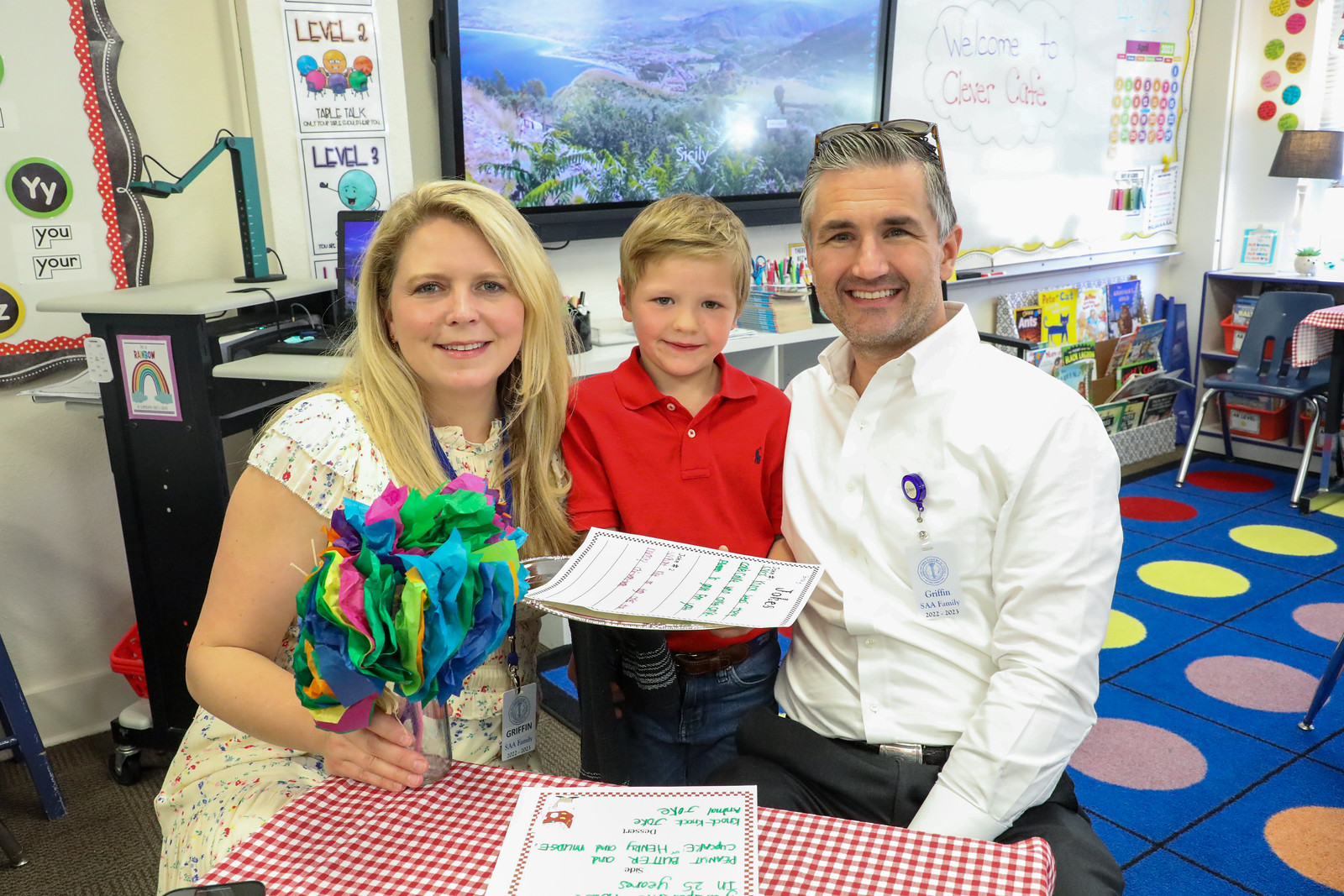In this vibrant and colorful photograph set in a preschool classroom, three individuals are kneeling and smiling directly into the camera. In the center is a young, blonde-haired boy, around three to five years old, dressed in a red polo shirt and blue jeans. Flanked on his left by a woman with long blonde hair and fair skin, who is wearing a white dress and holding a vase of tissue paper flowers, and on his right by a silver and gray-haired man in a white button-down shirt and gray slacks, with sunglasses perched on his head and a small beard visible. They appear to be proud parents, posing with their child likely after a classroom activity, as the boy holds up some papers he made. The room itself is lively, featuring a child-friendly carpet with multicolored circles, low bookcases, small child-sized chairs, and a whiteboard in the background with the words "Welcome to Clever Cafe." A table with a red and white checkered tablecloth sits in front of the group, displaying some handwritten notes or a certificate, further emphasizing the celebratory and educational atmosphere of the setting.